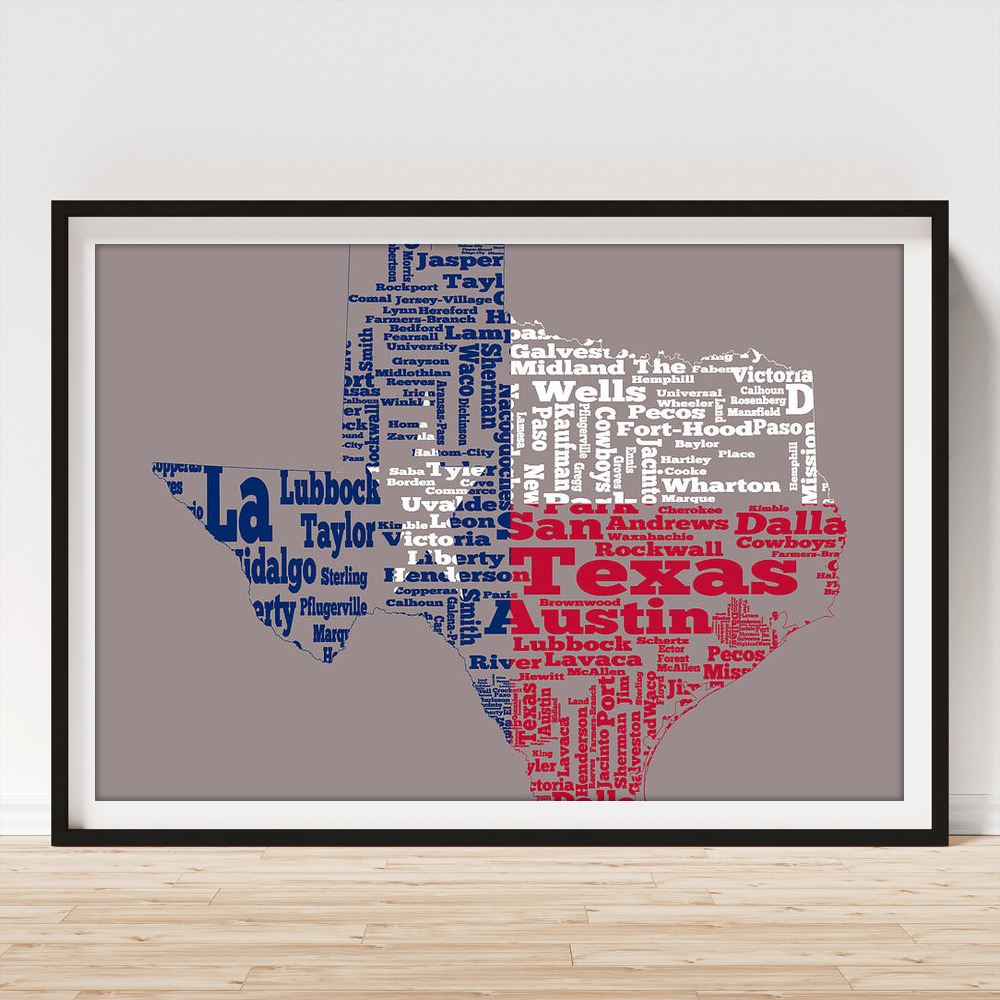This vertical rectangular image depicts a framed artwork leaning against a light gray wall on a light brown wooden floor. The frame is black with a white matting, encasing a painting with a gray background that features text forming the shape of the state of Texas. The text within the Texas shape is arranged in different sizes—small, medium, and large—and is colored blue, white, and red. On the left side of the state, the text is predominantly blue, with a white star composed of city names at the center. The top right portion of the state features white text, while the bottom right portion displays red text. Some of the visible city names include Dallas, Austin, Lubbock, Taylor, Sterling, Waco, Sherman, and Jasper. Prominent among the red text are the words "Texas" and "Austin." The entire composition merges geographic and typographic elements to artistically represent the Lone Star State.